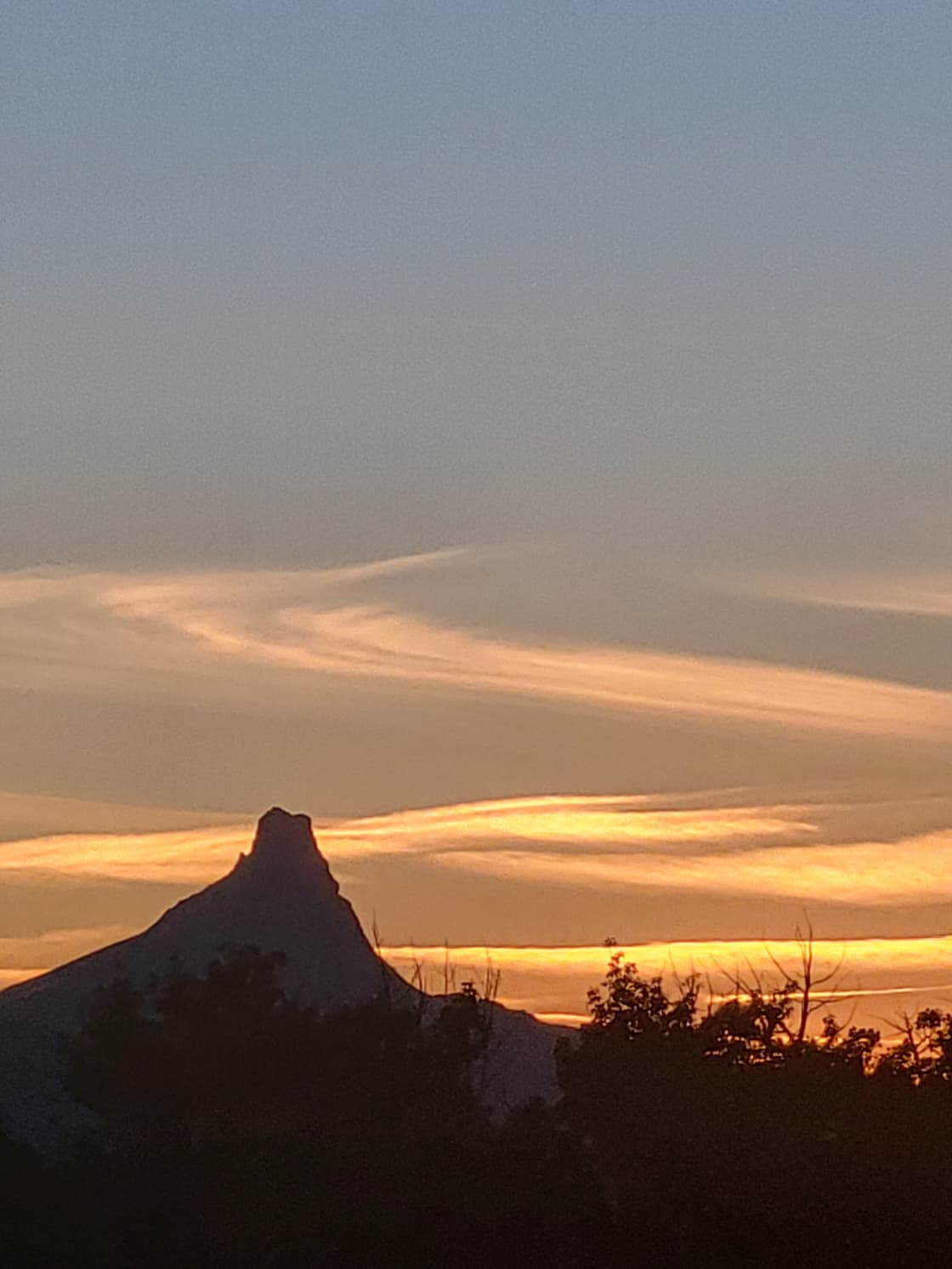This photograph captures the serene moment of a sunset, likely taken with a phone camera given its slight blurriness. The image is composed in portrait mode, making it a tall rectangle and emphasizing the vertical expanse of the sky, which constitutes roughly 70% of the frame. The sky transitions from a deep blue at the top to a vivid yellow along the horizon, indicative of the sun having just set. Wispy clouds, appearing like serpentine strokes of yellow and pink, meander across the scene. 

In the lower portion of the photograph, dark silhouettes of trees and shrubbery are prominently featured, appearing almost like black shapes against the bright background. The key focus, however, is a tall, distinctive mountain or butte with a slightly squared-off top, positioned off-center to the left. This landform rises sharply to its peak about a quarter of the way into the photograph before descending in a steep incline. The surrounding terrain and vegetation are enveloped in shadow, obscuring finer details but contributing to the stark contrast against the glowing horizon. The overall mood is accentuated by the interplay of light and shadow, capturing the fleeting elegance of twilight.